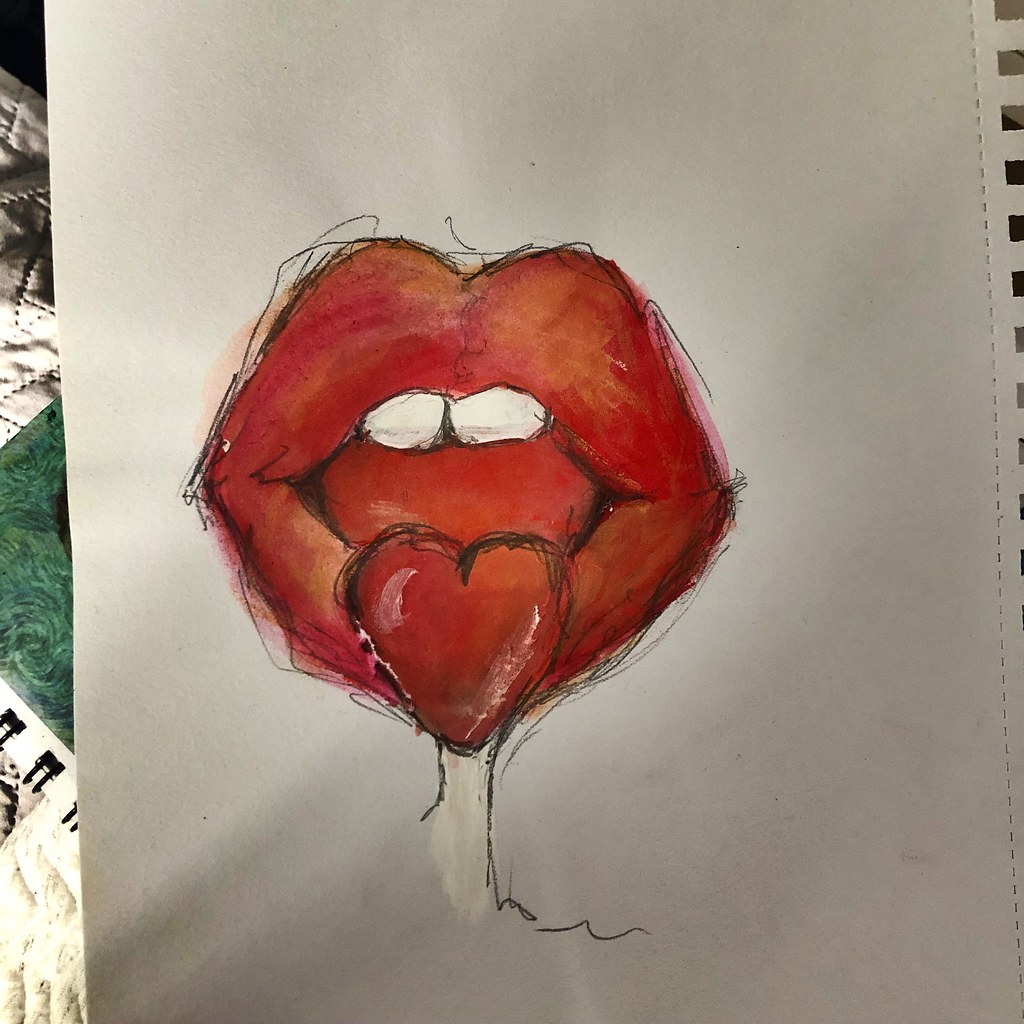This photograph showcases a detailed drawing on a white sheet of paper from a spiral sketching notebook. The focus is on a partially visible sketch page, with its perforated edges and spiral binding on the right suggesting it has been torn out from the notebook. The drawing itself depicts a mouth with large, red lips and two white front teeth. The tongue prominently extends and ends in a heart shape, both vividly colored in red. Black scribbles outline the lips and the heart, with additional scribbles trailing down from the heart. To the left, beneath the main sheet, part of another spiral notebook with a green and blue swirled cover and black spiral binding can be seen. The whole setup rests on a white quilt, its stitching subtly visible, adding texture to the scene.